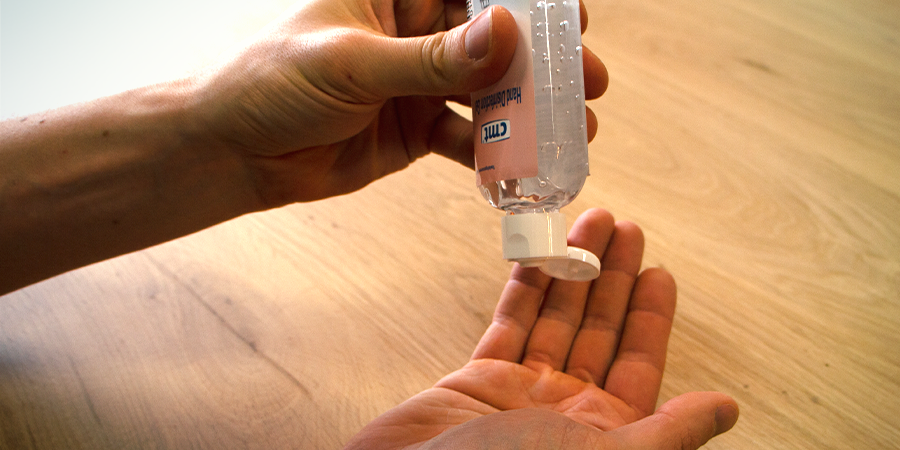The image depicts a person with a fair complexion and a couple of moles on their arm, about to use hand sanitizer. Their right hand is extended outward, palm up, positioned in the lower center of the frame, appearing ready to receive the sanitizer. The left arm, visible up to the forearm, extends from the left side of the image. The person grips a sample-sized, clear bottle of hand sanitizer—marked with a peach-colored label and black writing—in their left hand, thumb, and forefingers. The cap of the bottle is flipped open, indicating imminent use. The hand sanitizer inside the bottle is clear gel, visible with tiny bubbles. The background features diagonal light wooden flooring running from the bottom right to the top left, and a bright white light source is visible in the upper left corner.